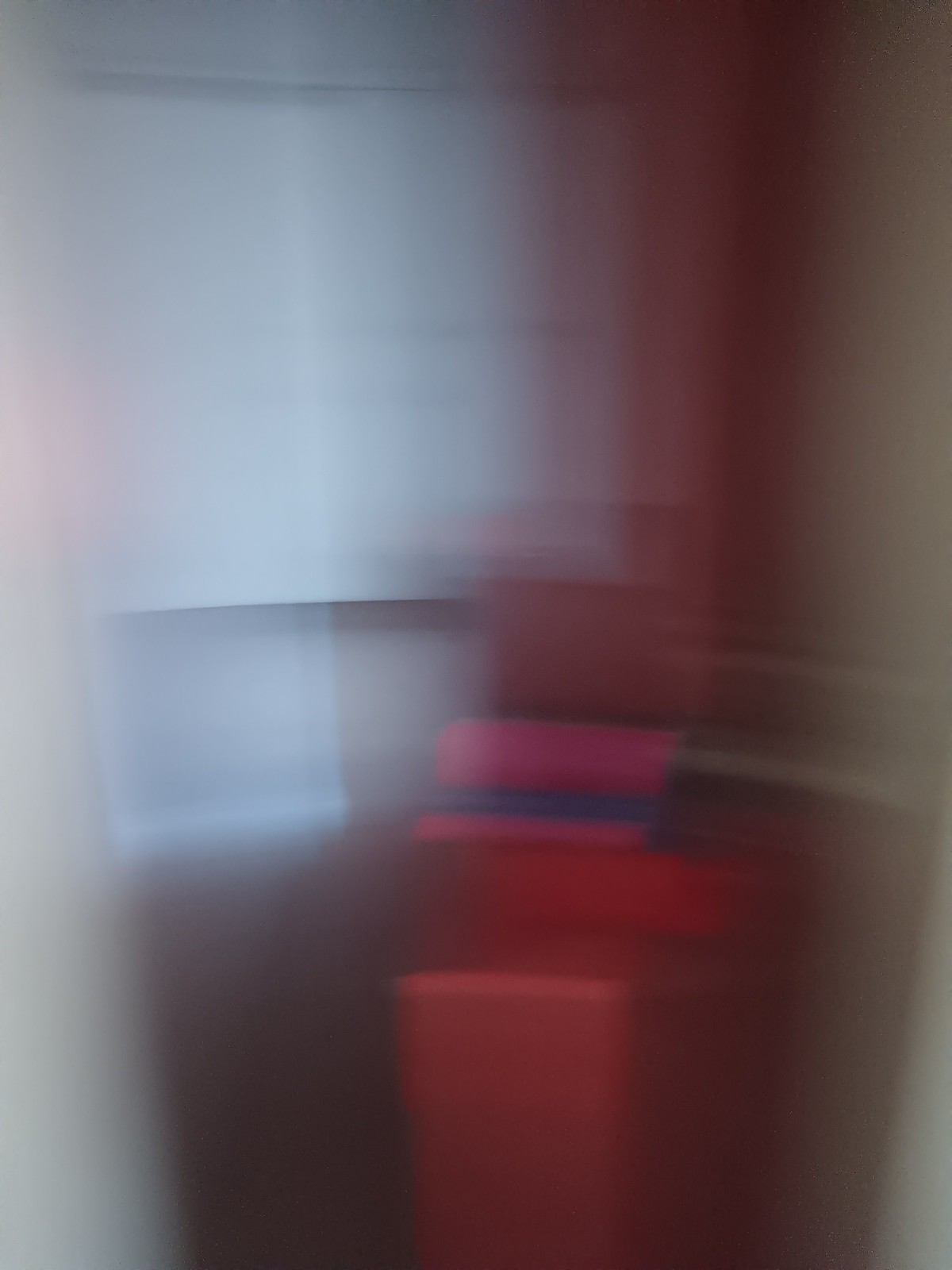This photograph appears to capture a scene in motion, resulting in a blurry and indistinct image. The left side of the photo is brightly lit, possibly by daylight or an artificial light source, while the right side is shrouded in shadows, suggesting an obstruction to the light. At the center of the image, there is a prominent red object, though its exact nature is unclear. It could possibly be a red hamper on the floor. The setting resembles an empty closet, evidenced by a potential clothes bar stretching horizontally across the middle. Draped over this bar is an indistinct object featuring pink and blue colors, contributing to the photograph's sense of disarray and motion. Above the bar, the image becomes even less discernible, with colors present but forms and details lost in the blur. The overall scene presents a contrast between light and dark areas, amplifying the mystery and ambiguity of the photograph's content.